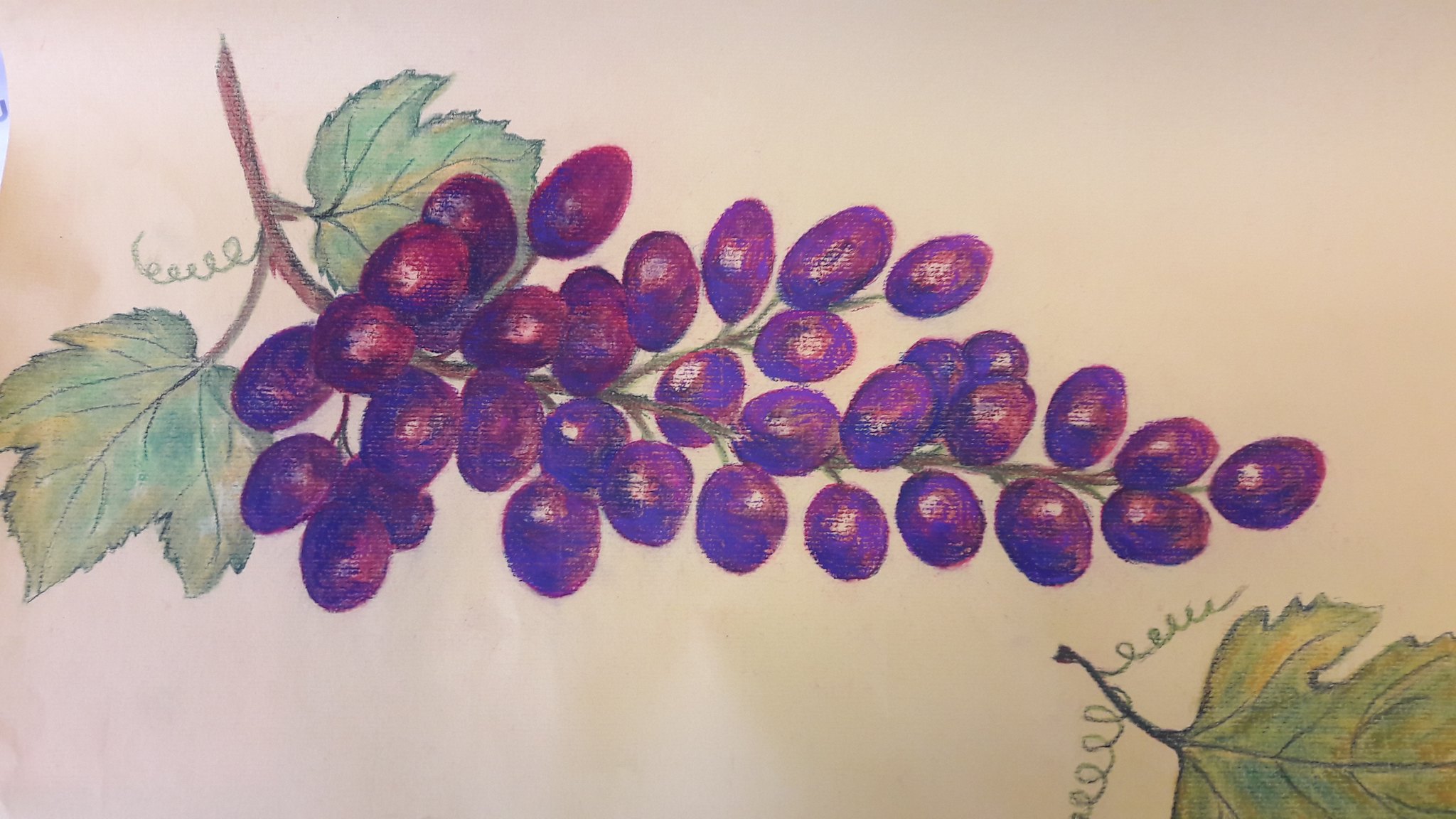A vibrant photograph captures a cluster of succulent, purple-hued grapes resting on a fabric-like tan background. The grapes glisten with a reflective sheen, highlighting their freshness. Surrounding the grapes are leafy green foliage with intricate veining, adding texture and depth to the composition. The brown stem from which the grapes dangle is clearly visible, enhancing the natural feel of the scene. Below the bunch, a green leaf with dark gray veining unfurls, accompanied by a whimsical corkscrew tendril extending from its stem. The detailed veining on the leaves and the interplay of light on the grape skins add a touch of realism and intricacy to this visually appealing image.